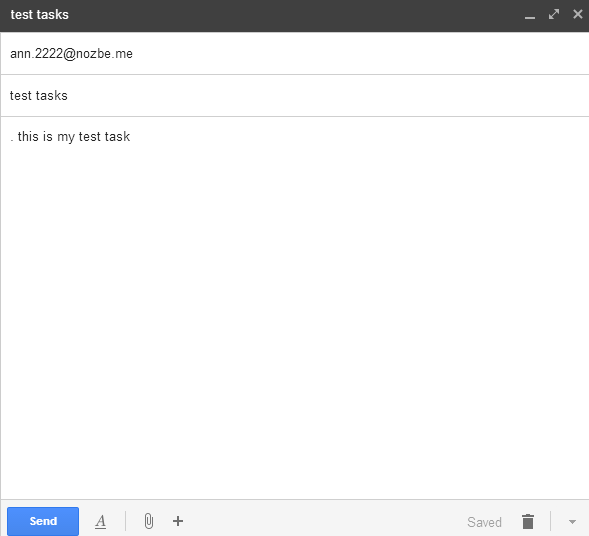This screenshot captures the Gmail compose window that appears when a user clicks on "Compose" in Gmail. The window is labeled "Test Tasks," which is displayed prominently in white text at the top. On the far right, standard window control icons for Minimize, Maximize, and Close are visible.

The email is being composed from the address ann2222@nozbe.me. The subject line reads "Test Tasks," and the body of the email is a brief message: "This is my test task." The setup suggests that the user might be utilizing this email for an automation workflow or a specific project, potentially triggering actions on the recipient's end upon sending.

No files or attachments are included in this email. At the bottom left corner, there's an option to send the message. The screenshot effectively illustrates the Gmail compose interface, highlighting specific details related to the email's content and potential use.